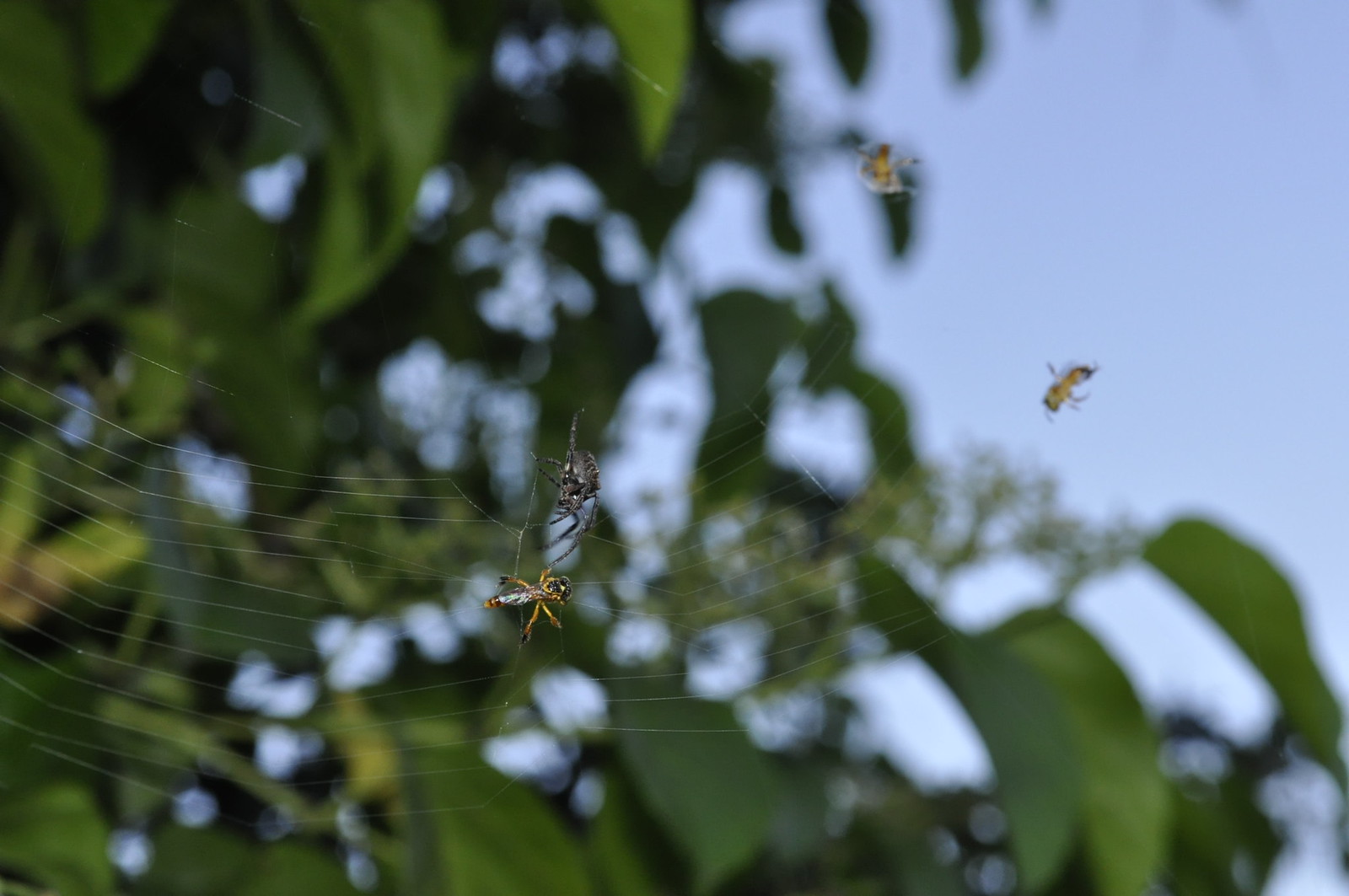In this outdoor photograph, the focus is on a spiderweb intricately woven among hazy, blurred trees and a pale blue sky background. At the center of the web, a black spider looms over its prey, a yellow-bodied insect with four small legs. Additional details reveal the presence of more insects caught in the web. To the right of the central pair, there are two more brown insects also entangled in the strands, seemingly reserved for later. The web itself spans horizontally from left to right and swoops upwards on the right-hand side, becoming more indistinct as it stretches outward. The overall effect highlights the meticulous and predatory nature of the spider’s world against a softly unfocused natural background.